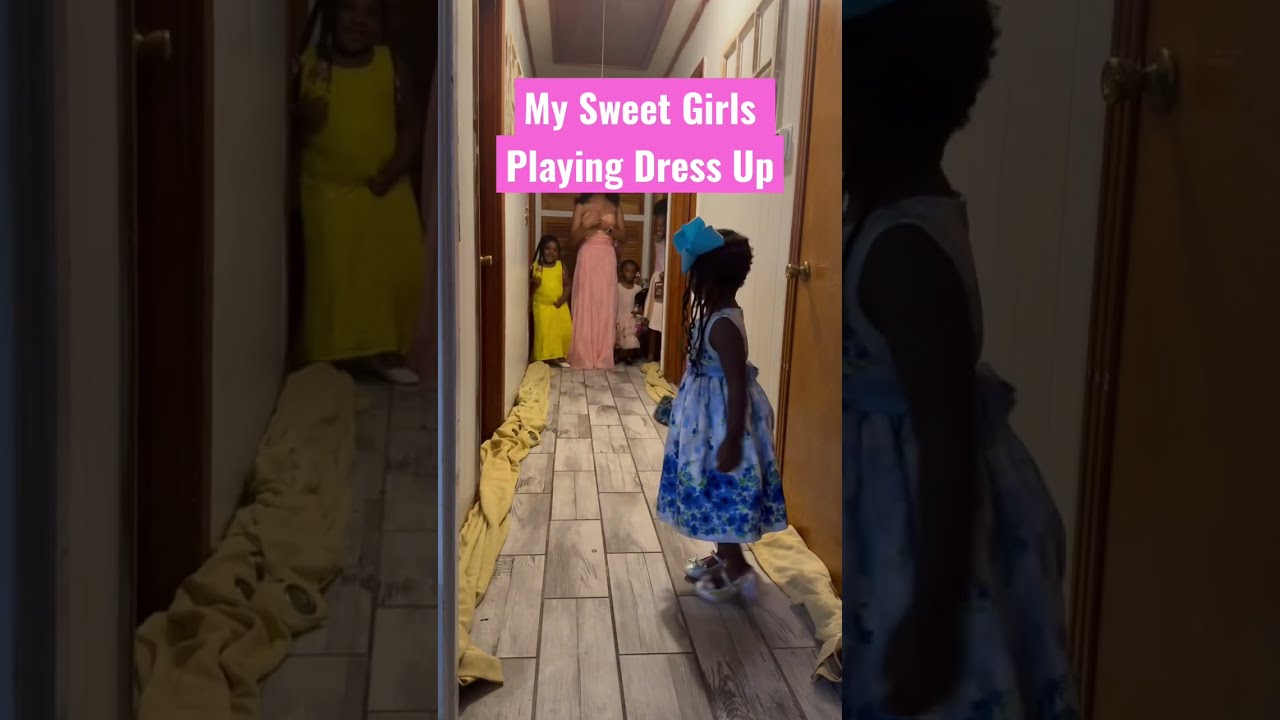In this vertically taken image, framed horizontally for a social media post, the central focus is a narrow, color vertical rectangle that features white text on a purple background saying, "my sweet girls playing dress-up." The scene is set in a hallway with white walls and brown doors, featuring wooden tiled floors. 

At the forefront is a little girl dressed in a blue and white floral dress with a large blue bow in her braided hair, and shiny white shoes. She is turned slightly, looking back toward the background. Further down the hallway stands a woman in a large pink dress, alongside three children: one in a yellow dress to her right, another in a white dress to her left, and a third in the foreground with blue and white floral patterns. Each side of the image contains blurry, close-up, darker renditions of the girls in the yellow and blue floral dresses, giving an impression of movement or a camera effect. This composition creates a joyful and intimate capture of a dress-up play session, reminiscent of a runway fashion show.